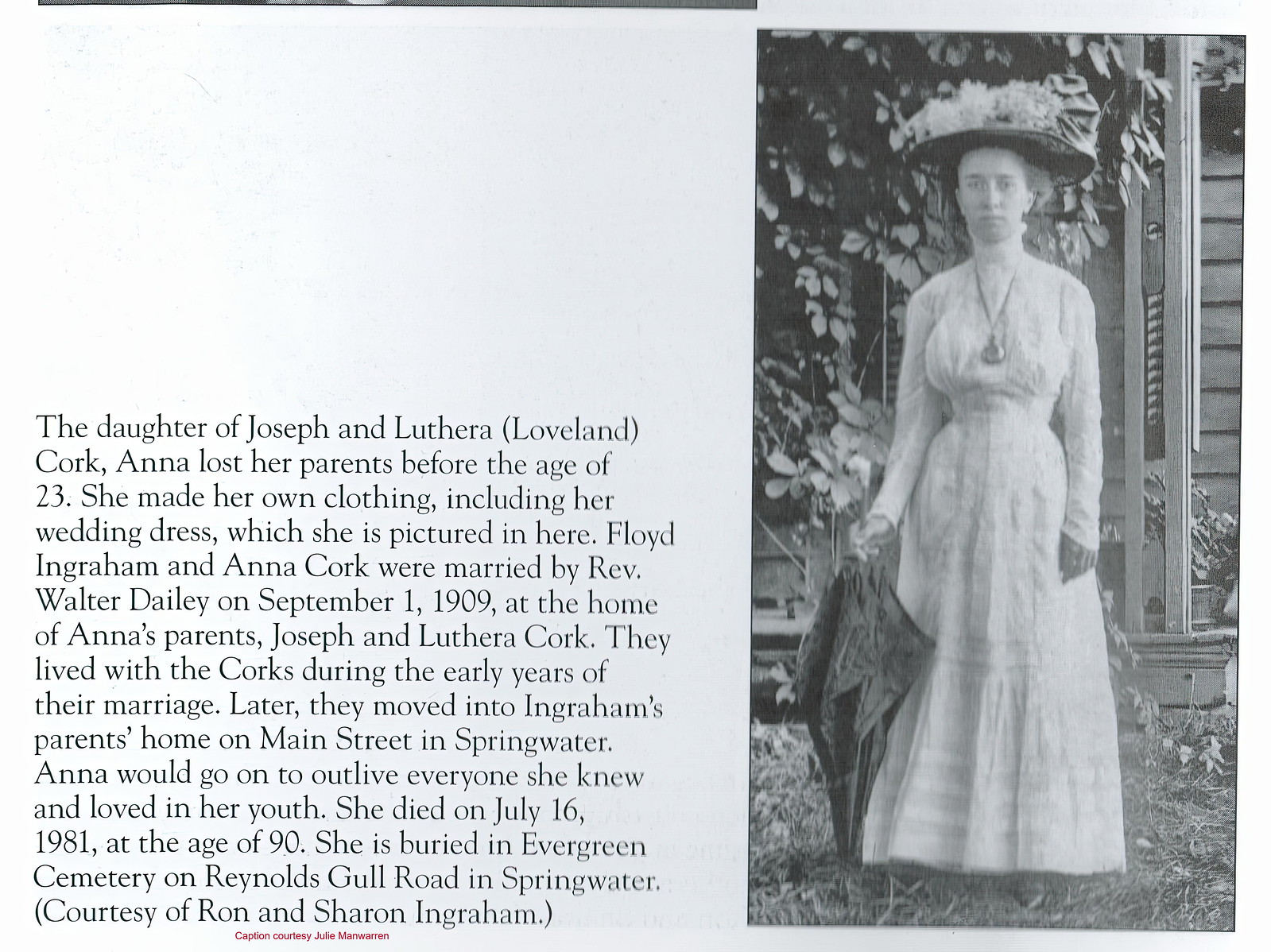This black and white photograph, appearing as part of an obituary from 1981, features Anna Cork in her handmade wedding dress from the early 1900s. The dress is a white, ruffled, and laced gown with a high collar, long sleeves, and a full-length skirt. She accessorizes with a large hat adorned with a bouquet of flowers and a prominent necklace. Holding a black umbrella down by her legs, Anna stands posed before a house with a large tree on a grassy lawn. The accompanying text reveals she was the daughter of Joseph and Luthera Loveland Cork. Anna tragically lost her parents before she turned 23 and crafted her own clothing, including the wedding dress she is pictured in. She married Floyd Ingram on September 1, 1909, in a ceremony officiated by Reverend Walter Daley at her parents' home. The couple initially lived with the Corks before moving to the Ingram family home on Main Street in Springwater. Anna outlived all her loved ones, passing away on July 16, 1981, at the age of 90. She is interred at Evergreen Cemetery on Reynolds Cole Road in Springwater, courtesy of Ron and Sharon Ingram.